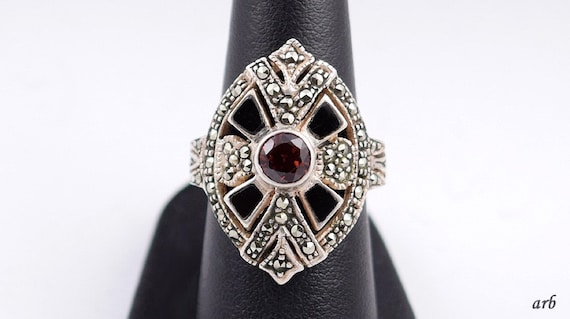The image showcases an advertisement for a jewelry store, featuring an ornate, vintage-style gold ring prominently displayed on a pitch-black mannequin hand against a solid white background. The ring is characterized by its detailed craftsmanship, marked by elaborate engraving and etching. Its oval shape is punctuated by a distinctive cross pattern, radiating from a large, deep red center gem, possibly a ruby. Smaller gems, possibly diamonds or similar stones, adorn the oval frame surrounding the cross. The cross's bars intersect the oval, creating a symmetric, balanced design. At the bottom right corner of the image, the letters "ARB" indicate the brand or creator of the ring. The ring's intricate details and vivid colors stand out sharply against the contrasting dark mannequin hand and plain white background, giving it a striking visual appeal.